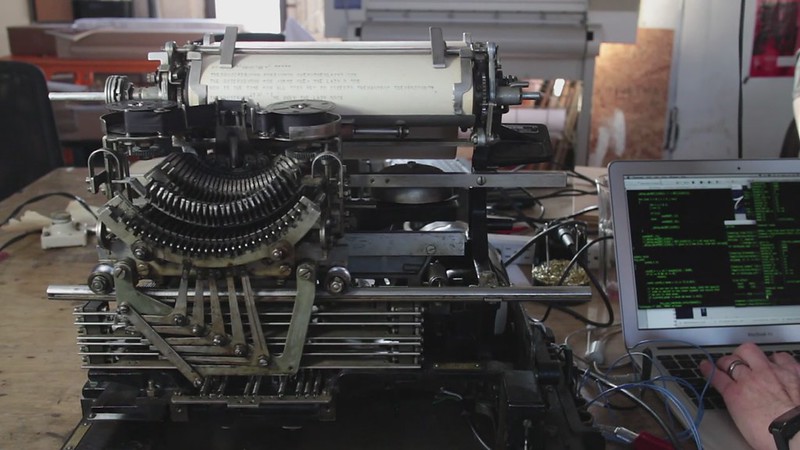A person is seated beside a modern computer and a vintage typewriter, likely from the 1920s or 1930s, identifiable by its old, worn keys and ribbon. This unique setup suggests the individual may have integrated modern technology with the manual typewriter, perhaps for a specialized task. They are in an industrial setting, possibly a machine shop or print shop, as indicated by the massive rolls of paper and a white printing device visible in the background. Sunlight streams through windows, illuminating the scene. The person, adorned with a wedding ring and a watch, exudes a blend of old-world charm and contemporary flair. The computer screen displays text that is unreadable from this perspective.